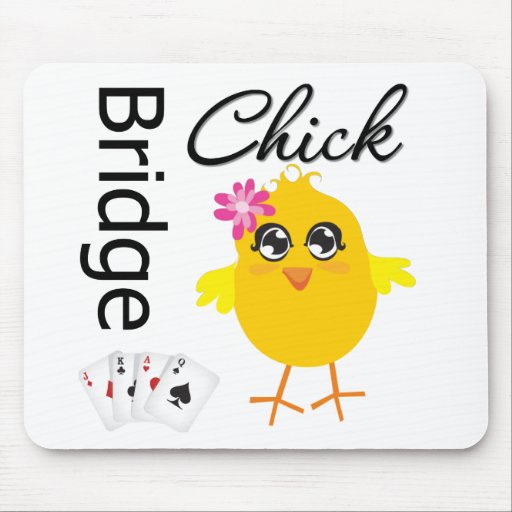The image showcases a drink coaster with a gray wood-stained background. Predominantly in the center, there is a rounded white square covering most of the image. Depicted on the square is a vivid cartoon representation of a gold-colored chick. The chick has large, exaggerated black eyes with eyelashes, a small orange beak, and orange feet. A small pink flower adorns the left side of its head, contributing to its charming appearance. Above the chick, the word "chick" is inscribed in large black cursive letters. Running vertically from the top to the bottom of the square on the left, the word "bridge" is written in bold black block letters. Below this text, four cartoon cards are fanned out, displaying the jack of diamonds, king of clubs, ace of hearts, and queen of spades. This detailed and whimsical design suggests that the coaster is an affectionate tribute to female fans of the card game bridge, making it a perfect accessory for a bridge enthusiast's wall or desk.